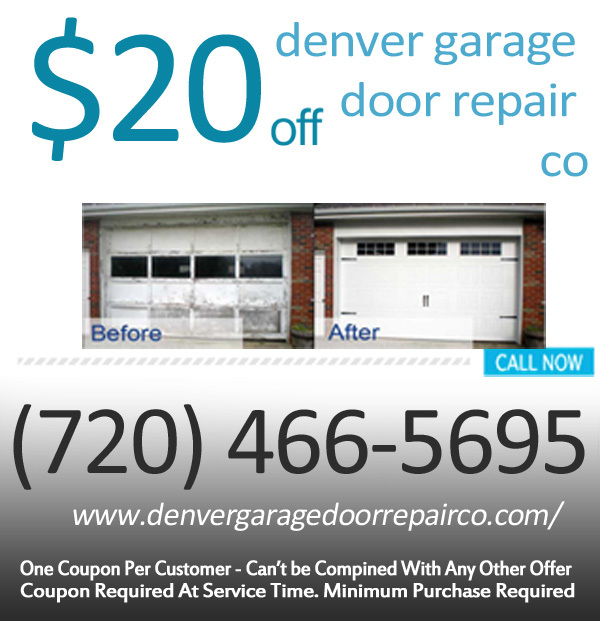**Caption:**

The image displays a promotional advertisement for Denver Garage Door Repair, featuring a "$20 Off Denver Garage Door Repair" offer prominently at the top, with "CO" hinting at the location. The visual showcases a remarkable transformation with a before-and-after comparison: the "before" picture reveals a dilapidated, grimy, and barely functional garage door, while the "after" picture highlights a pristine, new white garage door that appears sturdy and effortlessly sleek. Additionally, the corner of the image encourages viewers to "Call Now" with the provided phone number, 720-466-5659. At the bottom, the company's website, www.denvergaragedoorrepairco.com, is listed alongside detailed offer terms stating, "One coupon per customer, can't be combined with any other offer, coupon required at service time, minimum purchase required."